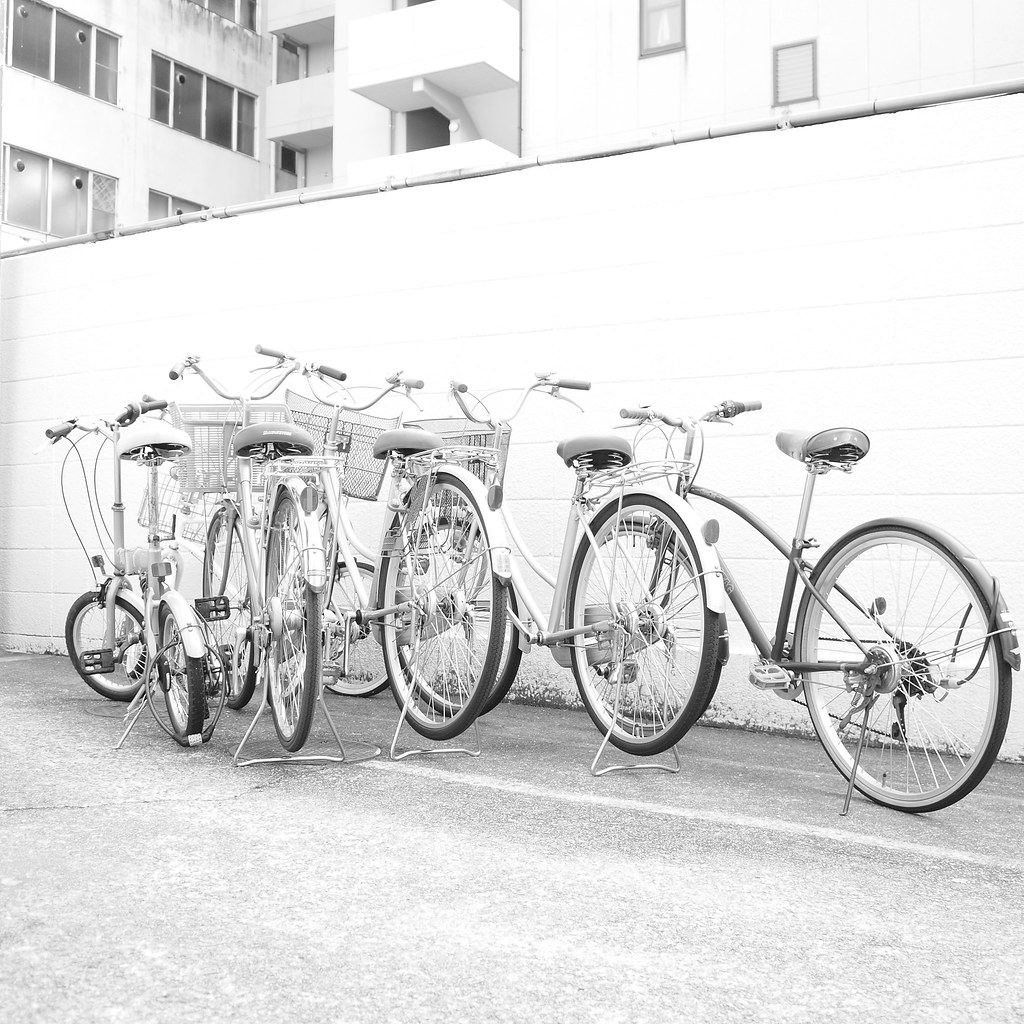This black-and-white photograph captures a row of five bicycles neatly lined up on a light grey cement road. Four of the bicycles are old-school, beach cruiser style, each equipped with front baskets and a silver kickstand propping them up. Beside them stands a more modern bicycle, noticeably smaller and without a basket. The bikes feature light grey frames, with silver-white spokes and dark brown tires, and white brake cables running to the handlebars. Directly behind the bikes is a six-foot-tall white brick or concrete wall. The scene extends beyond the wall, revealing parts of a light-colored building with signs of rust, glass windows, and white balconies, suggesting it could be a condominium or apartment complex. The nostalgic feel of the retro bicycles aligns with the timeless quality of the monochrome image.